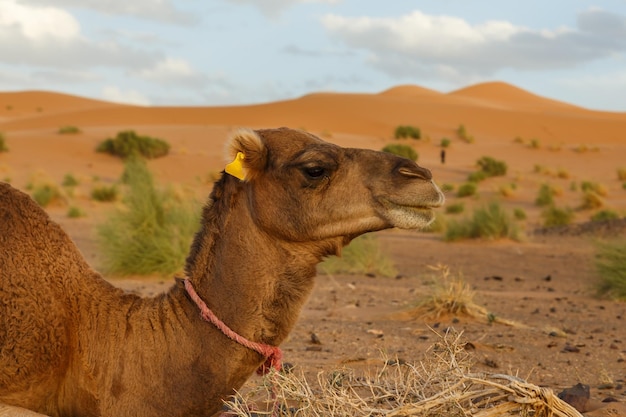This detailed photograph captures a camel lying on the sandy, dry ground of a desert landscape. The camel, with its tan, camel-colored brown coat, sports a light red rope necklace around its neck and has a yellow identification tag in its ear. Its large head features round, small ears, and its mouth is closed in a composed expression. Only the initial curve of its large hump is visible, suggesting the rest of its body is obscured as it lies on the ground. Surrounding the camel, the ground is strewn with dead plant materials, including white, spiky branches. In the background, towering sand dunes rise, interspersed with sparse desert shrubs and green vegetation, all under a partly cloudy sky. The landscape further away includes sand-covered mountains, offering a fitting habitat for the camel. The overall scene combines elements of the camel's appearance and the arid environment, capturing the essence of desert life.